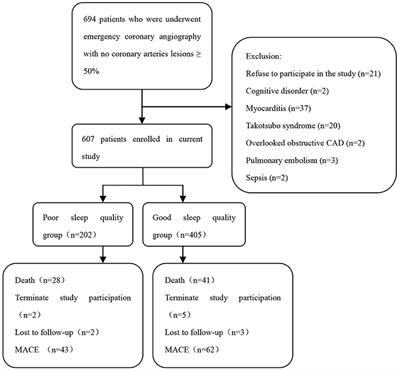This vertical flowchart diagram, predominantly black and white with a notable pink box, visualizes a study involving patients who underwent emergency coronary angiography. At the top, a rectangular box labeled "694 patients who underwent emergency coronary angiography with no coronary artery lesions (50%)" leads via a downward arrow to another box labeled "607 patients enrolled in current study." From this central box, an arrow extends to the right, connecting to a larger box containing exclusion criteria with details such as refusal to participate (N=21) and various medical conditions including cognitive disorder (N=2), myocarditis (N=37), Takotsubo syndrome (N=20), overlooked obstructive CAD (N=2), pulmonary embolism (N=3), and sepsis (N=2).

The central box also points downward to two smaller boxes: the left one labeled "Poor sleep quality group (N=202)" and the right one labeled "Good sleep quality group (N=405)." Both groups further branch out into two larger rectangles below. The left group's larger box indicates outcomes like "Death (N=28)," "Terminate study participation (N=2)," "Loss to follow-up (N=2)," and "MACE (N=43)." Similarly, the right group's box lists "Death (N=41)," "Terminate study participation (N=5)," "Loss to follow-up (N=3)," and "MACE (N=62)." Each box is connected by black arrows, clearly mapping the flow of data through the study's stages and outcomes.